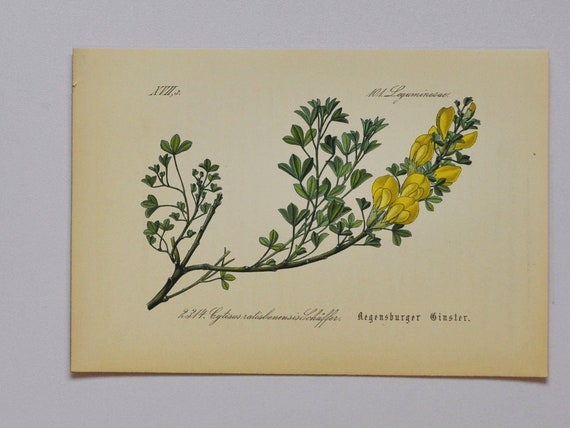This illustration, likely a vintage botanical print or card, features a beautifully detailed depiction of a flowering branch on a slightly yellowed, beige background with aged edges, evoking a timeless quality. The main branch ascends from the left side of the composition and bifurcates into two offshoots. The left offshoot is adorned with lush green leaves, while the right offshoot extends further and is bedecked with clusters of round, yellow flowers and smaller buds in various stages of bloom. Notably, the illustration includes textual elements: at the top left, there is an inscription that reads "XVII" followed by an unreadable notation, and beneath the flowers, a partially legible signature with an 'L'. The bottom of the card exhibits a lengthy, complex Germanic script, possibly indicating the scientific name, although much of it is difficult to decipher. The text includes phrases like "Regensburger Ginster" or similar, suggesting the specific categorization of the plant. The overall effect is a precise, aesthetically pleasing image capturing both the botanical features and informative context of this flowering branch.